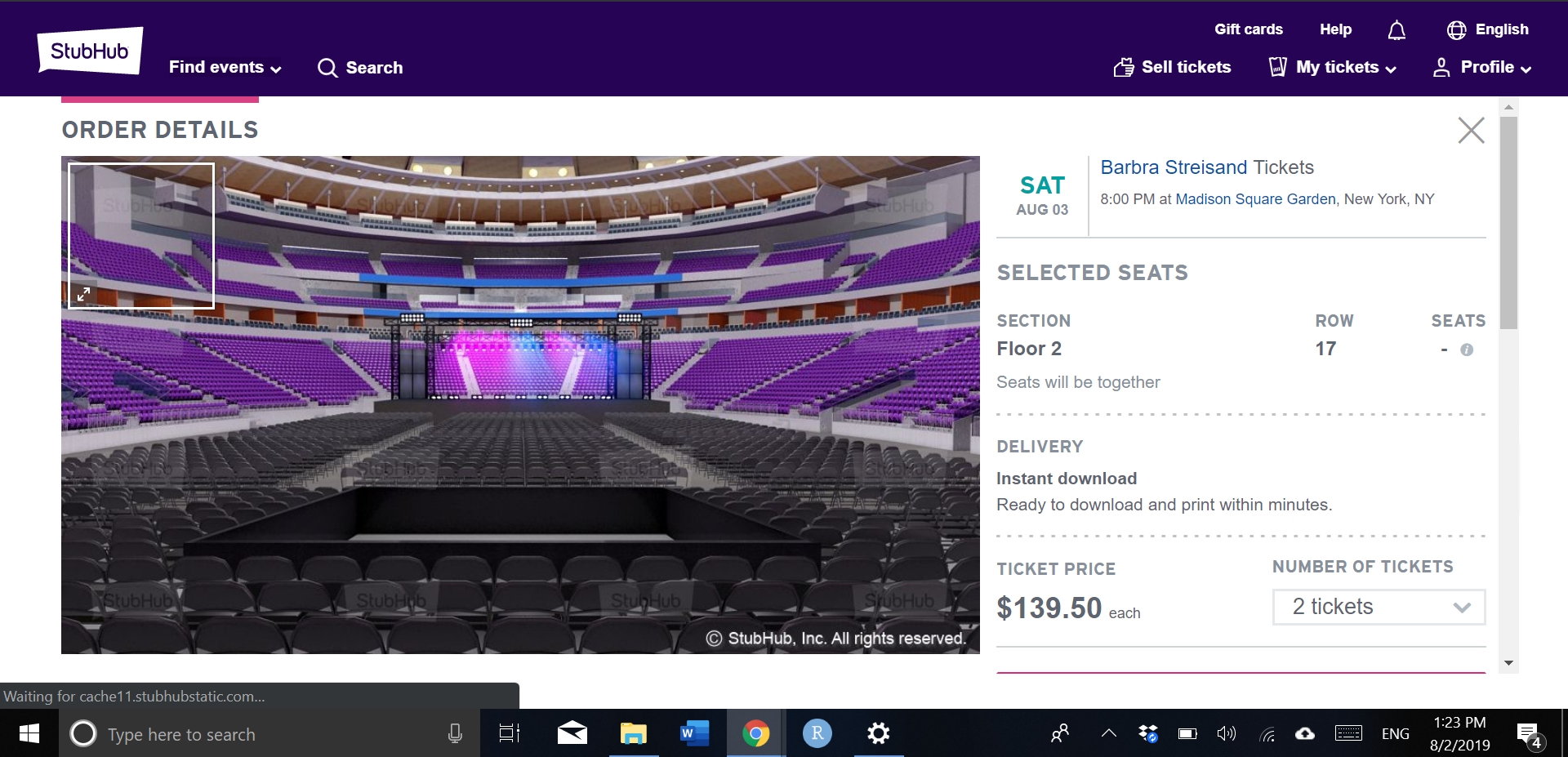This image showcases the StubHub website interface. The top navigation bar is a rich dark purple shade. Positioned on the left side is the StubHub logo, featuring dark purple text with a white background. Adjacent to the logo, there is a drop-down menu labeled "Find Events," followed by a search bar for user convenience. 

On the right side of the top bar, there are several options: "Gift Cards," "Help," a bell icon for notifications, and a language selection option displayed as "English." Below these, there are drop-down menus for "Sell Tickets," "My Tickets," and "Profile."

The main section of the webpage has a clean white background. It prominently features the header "Order Details." Beneath this, there is a virtual seating chart image of the concert venue, allowing users to visualize the location of their seats. 

To the right of this seating chart, detailed information about the concert is provided. It indicates the event details as follows: "Saturday, August 3rd, Barbra Streisand, 8 PM at Madison Square Garden, New York, New York." The selected seats are specified as "Section Floor 2, Row 17," with a note that the seats will be together. 

Further details include the delivery method, stating "Instant Download," available for downloading and printing within minutes. The ticket price is listed as "$139.50 each," and the total number of tickets is two.